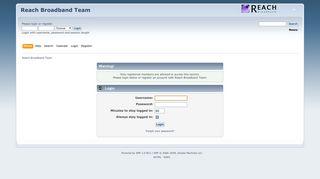In this screenshot, the heading "Reach Broadband Team" is prominently displayed in the upper left-hand corner, with the Reach company logo situated in the upper right-hand corner. Below this, on the left side, there are two text boxes and a dropdown menu, though the text within these elements is too small to discern. On the far right of this section, there appears to be another text box, which likely functions as a search bar. 

Further down on the left, there are six buttons, with the first button highlighted by an orange rectangle. Separating these elements from the lower section is a dark gray line that spans horizontally across the image. Beneath this line, some text is visible on the left side. Centrally aligned, there are two distinct sections: the upper section contains some illegible text, while the lower section includes fields for a username and password, as well as additional smaller input boxes whose purpose is unclear. Below these fields, a central button labeled "Log In" is clearly visible. At the very bottom of the image, two additional lines of text are centered.